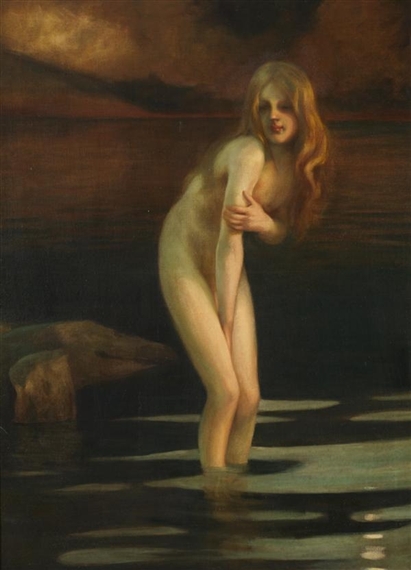This detailed painting portrays a young naked woman standing ankle-deep in dark, reflective water. Her long, wavy hair, a blend of reddish, blonde, and brown hues, cascades over her shoulders, adding a touch of softness to the scene. The woman is slightly hunched over, exuding an aura of shyness and vulnerability. She covers herself with her right arm extending down to almost kneel level, while her left hand gently grasps the upper arm, shielding her chest. Her face, partly in shadow, is turned away from the viewer, with her eyes seemingly a bit closed or looking downward, creating a sense of introspection. Reddish lips add a subtle hint of color to her otherwise neutral-toned complexion. 

The water around her is dark and moody, with reflections that add depth to the scene, complemented by small rocks visible in the bottom left corner. The atmospheric tones of the background blend shades of dark, reddish, orangish, and black, enhancing the painting's introspective and slightly melancholic mood. The overall color palette is dominated by tan and neutral brown hues, imbuing the image with a timeless quality, reminiscent of classical artworks, such as Botticelli's "Birth of Venus." Despite the intricate details, there is no visible artist's signature on the painting.